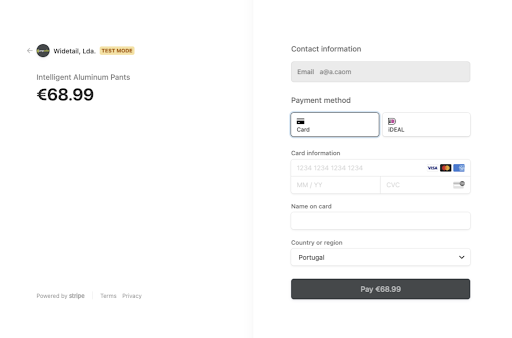The image depicts a webpage from the company "Wide Tail Limited" showing a test mode for purchasing intelligent aluminum parts priced at €68.99. The prominently featured page has red lettering with a highlighted yellow banner displaying the product name and price. On the right side of the webpage, contact information is provided in a blue box where users enter their email addresses and select a payment method. Available options include using a credit card or the iDEAL payment system. 

Below the contact information, users can input their card details in white text fields, including the credit card number, expiration month and year, the CVV number, and the cardholder’s name. Additionally, there is a dropdown menu for selecting the country or region.

At the bottom of the form, a thick black box prominently displays the total amount of €68.99, reassuring the user of the price they are about to pay. Upon completing the form, users would click this box to proceed with the purchase, which likely navigates to a subsequent page for shipping details.